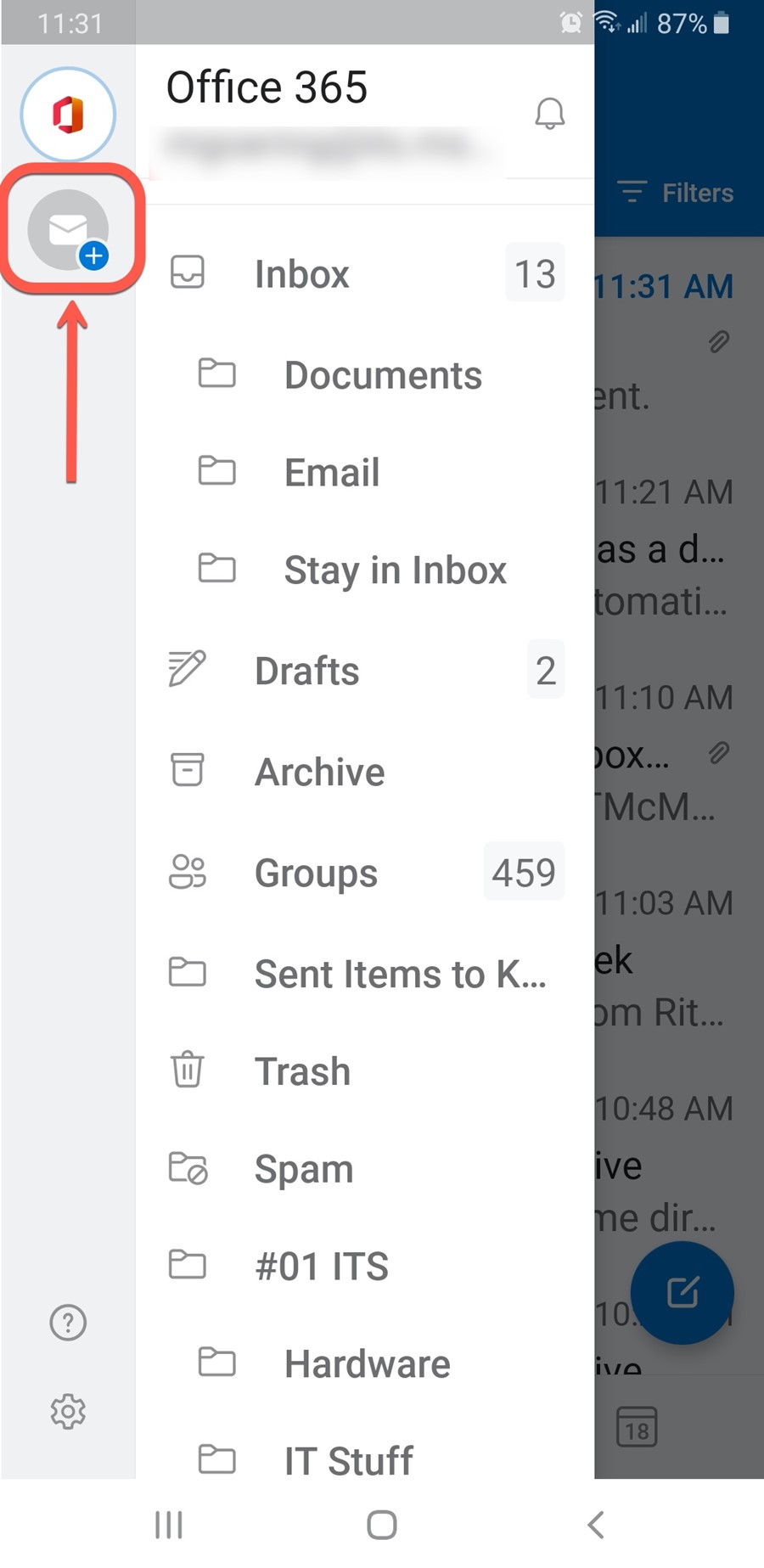Screenshot of a user's phone displaying their Office 365 email inbox. The phone's status bar at the top indicates the time is 11:31, with the battery level at 87% and the internet connectivity icon visible on the right. 

The primary screen shows the Office 365 email application. To the left, a sidebar reveals the email folders and various categories, including:
- A red circle or oval icon at the top.
- A red box with a red arrow around an envelope icon, indicating something important.
- Categories such as "Inbox" (13 emails), "Documents," "Email," "Stay in Inbox," "Drafts" (with 2 items), "Archive," "Groups" (459 items), "Sent Items" (K...), "Trash," "Spam," "Number sign #0," "IT Support," "Hardware," and "IT Stuff".

The right side of the screen is slightly darkened, displaying the right panes of emails, primarily showcasing their timestamps. In the background, the interface reveals a mix of various email-related icons and options, with some personal information redacted for privacy.